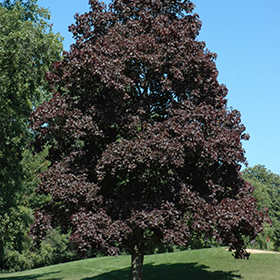This small square photograph captures a magnificent, large deciduous tree adorned with deep, dark purple leaves. The tree is incredibly full, with branches and limbs that stretch nearly to the ground, casting a distinct shadow on the perfectly mowed grassy area beneath it. Although the very top of the tree is not visible in the photo, the triangular shape of the foliage and the partial view of the trunk are prominent. The tree stands proudly on the side of a low hill, surrounded by green trees lining the grassy expanse to the left. In the background, a beautiful, cloudless blue sky accentuates the vibrant scene. To the right, the tops of smaller green trees are visible. The tree has a slightly bare spot in the middle, allowing the bright blue sky to peek through. This picturesque setting captures the lush, luxurious beauty of the tree, with its purple leaves contrasting sharply against the vivid greens and blues of the landscape, creating a truly enchanting image.